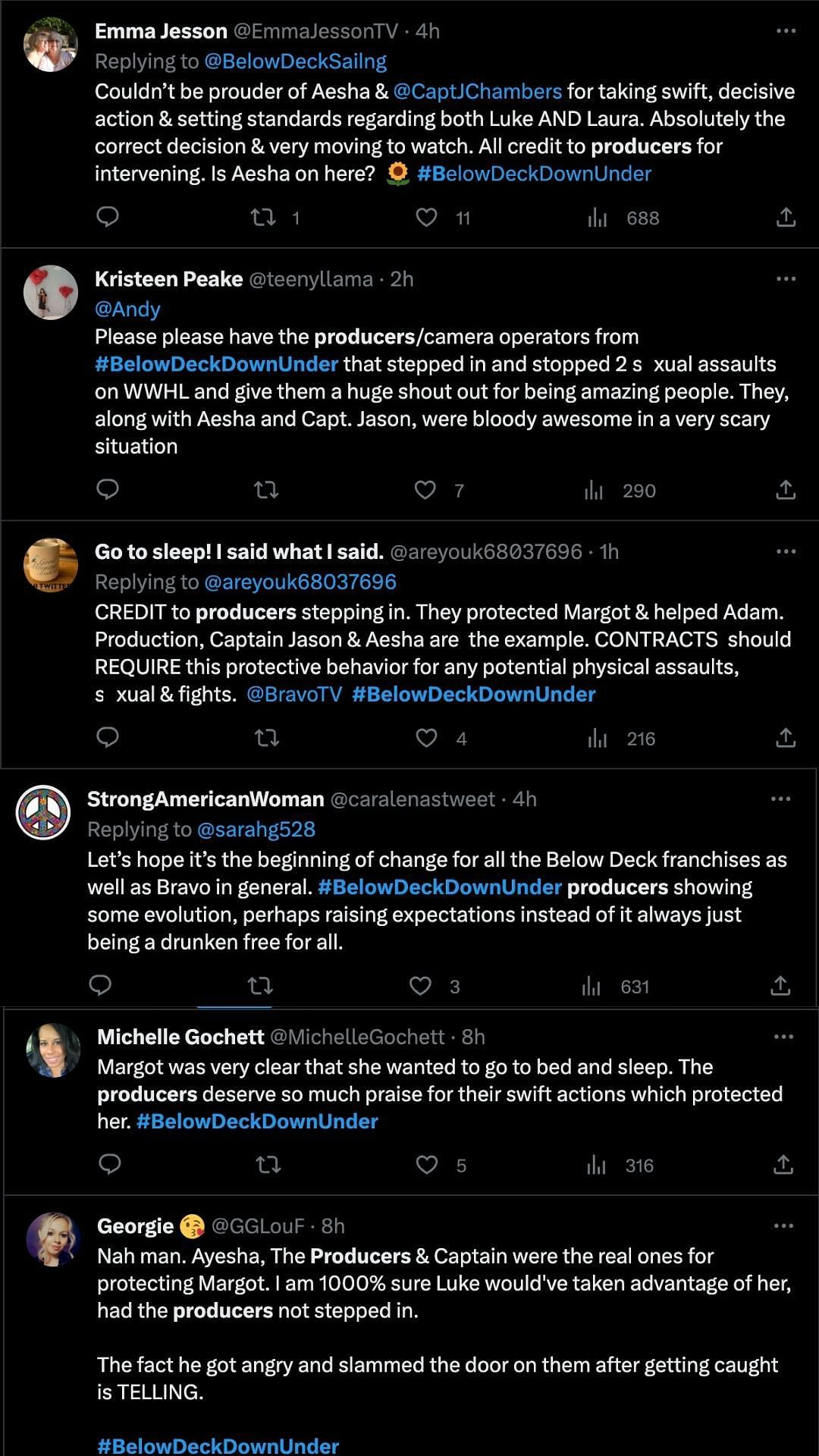**Caption:** Screenshot of a Twitter conversation with a black background. At the top is Emma Jensen's tweet replying to Below Deck Sailing, written in white text: "Couldn't be prouder of Ashia and Captain Hugh Chambers for taking swift, decisive action and setting standards regarding both Luke and Laura. Absolutely the correct decision and very moving to watch. All credits to producers for interviewing." It continues to mention "Ashia" and references "Below Deck Under."

Following this, Christine Peak replies, urging recognition for the production camera operators from "Below Deck Down Under" who intervened to stop two sexual assaults. She praises their bravery, along with Ashia and Captain Jed, for their commendable actions during a frightening situation.

The screenshot shows a thread with six nested conversations, ending with "#BelowDeckDownUnder" in blue at the bottom.